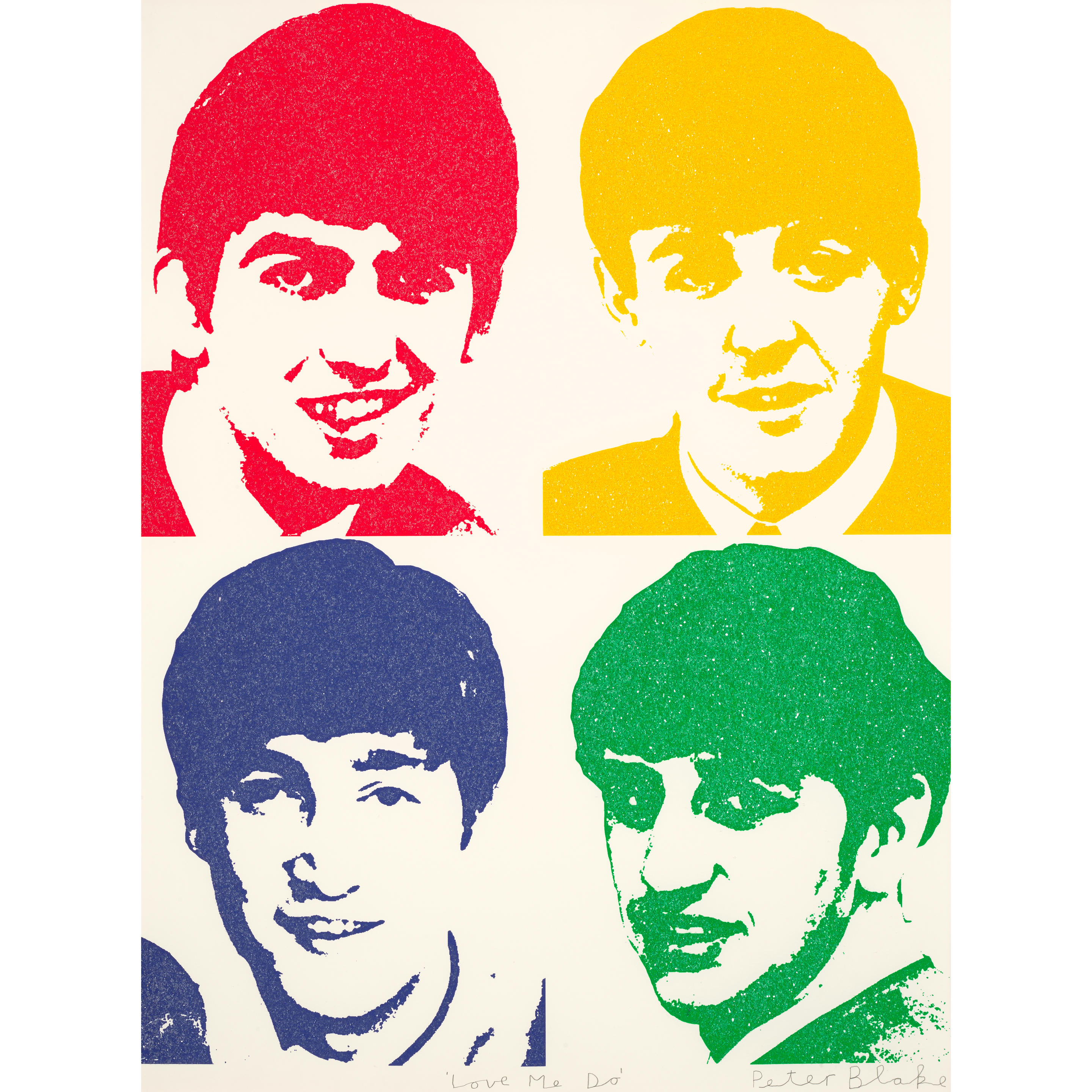This image is a vibrant and artistic tribute to The Beatles. The artwork, signed in cursive by Peter Blake at the lower right-hand corner, features a mix of vivid colors and eye-catching composition. The piece includes four distinct portraits of the band's members, each rendered in a different hue and style. The first portrait on the left is done in red, showing the subject looking directly at the viewer. The top right portrait is a yellow silhouette, while the bottom left is depicted in blue. Next to the blue portrait, the subject is shown in green with all figures except the last one portrayed from a head-on perspective. The final figure on the right is turned to the side but still meets the viewer's gaze with a full-face view. At the bottom of the artwork, the phrase "Love Me Do," a nod to one of The Beatles' famous songs, is written in pencil. This detailed and colorful homage captures the essence of The Beatles, even if the specific members' identities aren't immediately recognizable to the casual observer.